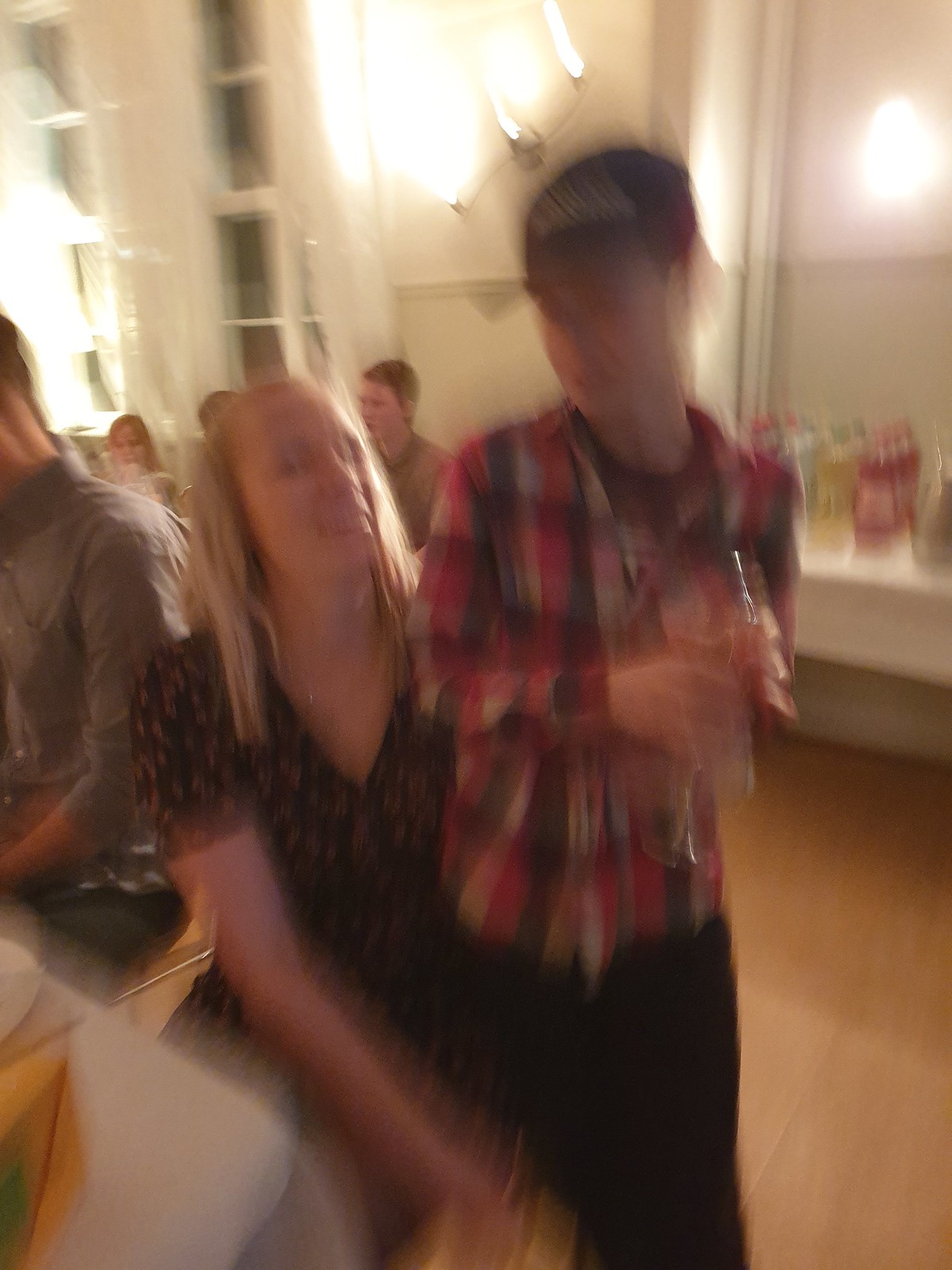The colour photograph depicts a blurred yet vibrant scene of a celebration or party in a function hall. In the foreground, a blonde-haired woman dressed in a black floral-print dress is seated at a table covered with a white tablecloth, smiling at the camera. To her right stands a young man, possibly her son, wearing a red, black, and white checkered shirt over a black and white t-shirt, with black bottoms and a cap. He is holding two glasses, though their contents are indistinguishable. The man's face is notably blurred, suggesting motion during the capture. 

Behind them, the table is laden with large two-litre bottles of various coloured beverages, such as pop or fruit drinks, lined up in multiple rows. More individuals are visible in the background, adding to the bustling atmosphere. The hall features sconce lights on the walls, with their overexposed white streaks indicating the camera moved during the shot, contributing to the overall blur. The room appears well-lit, with possibly hardwood floors and two large windows contributing to the lively environment. 

The blurred motion captured in the image gives it a ghosted, elongated appearance, adding a dynamic feel to the festive scene.